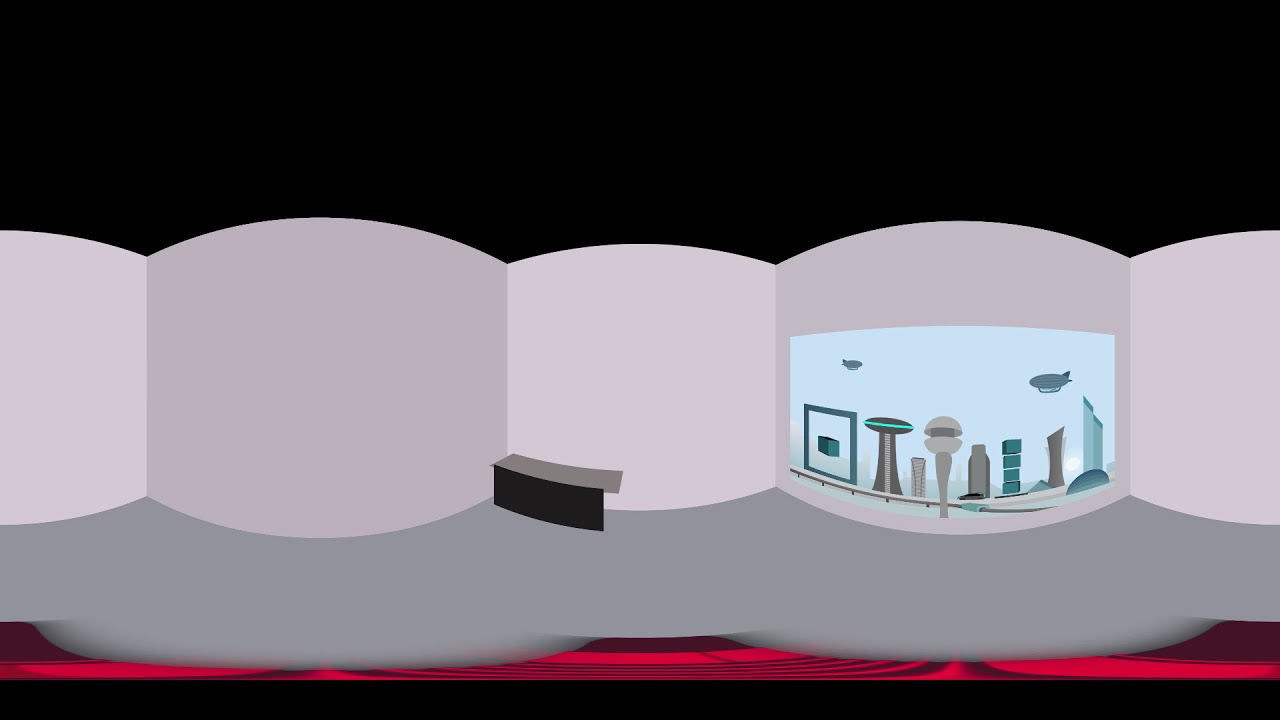The image is a computer-generated design of an ultra-modern, possibly futuristic room, featuring a series of interconnected curved walls that run horizontally across the center. The walls are rendered in varying shades of light gray, creating a dynamic, flowing landscape that bulges and flattens rhythmically. In the indentation between the curved and flat sections of the wall, there is a small black bench. To the right, one of the curved walls prominently displays what may be a painting or window, showcasing a sci-fi cityscape. This cityscape features a light blue sky filled with spaceships and a collection of seven tall, thin skyscrapers with uniquely shaped tops, such as an oval or an arch turned upside down. The floor beneath these structures is a darker gray with a hint of red, adding depth to the scene. The overall composition gives off a vibe of a dystopian art gallery, with the top part of the image remaining starkly black, framing the intricate details below.